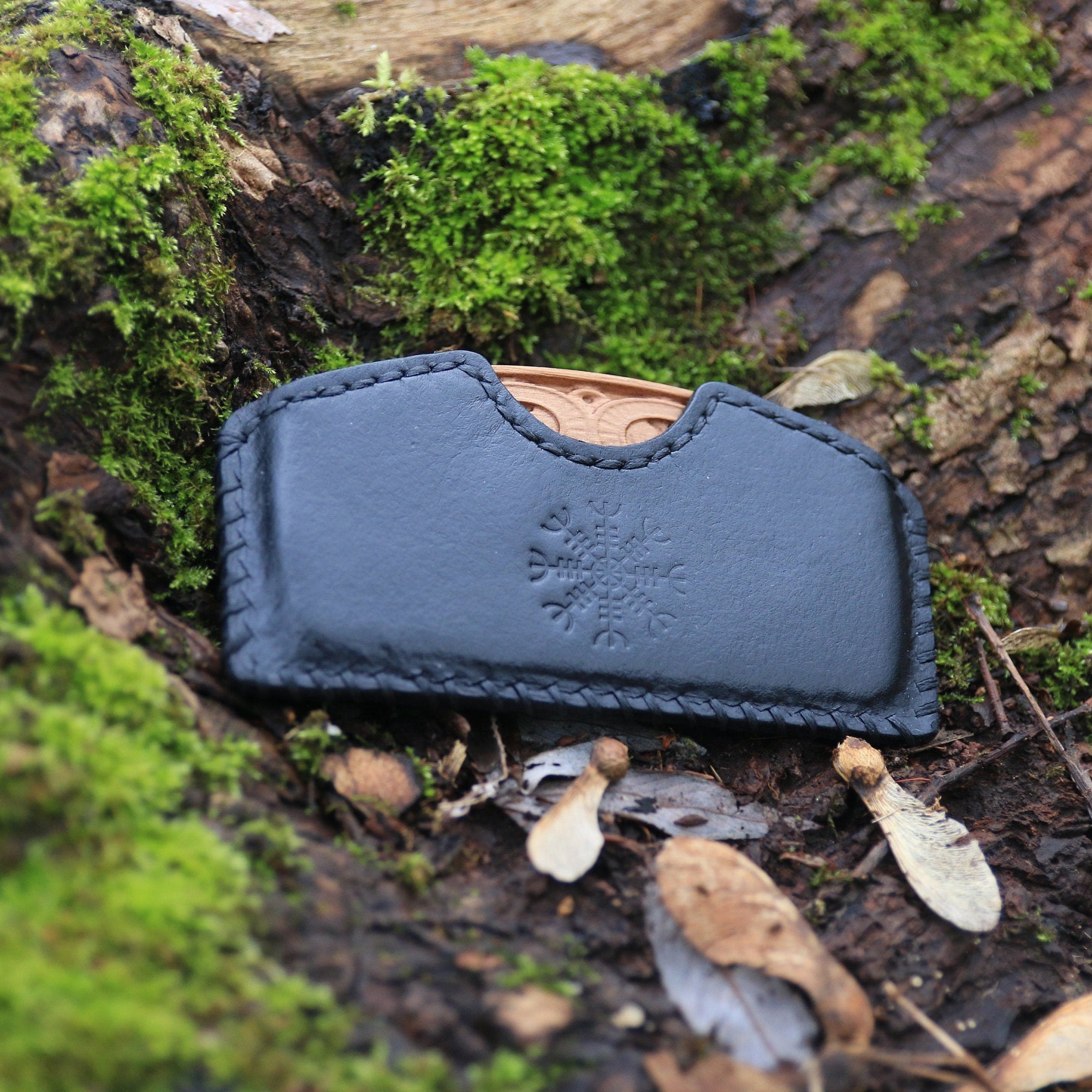The image features a black leather sheath set in a dirt trough amidst a forested area. The sheath is adorned with intricate stitching along its edges and features an embossed snowflake design on the front. This design consists of a central circle with eight radial lines, each flanked by three smaller lines and ending in a U-shaped curve. Inside the sheath, a light tan, possibly plastic, object with curved edges is partially visible. The scene around the sheath includes patches of moss and small plants, as well as scattered dead leaves and dark brown mud, contributing to the forest floor's natural look.